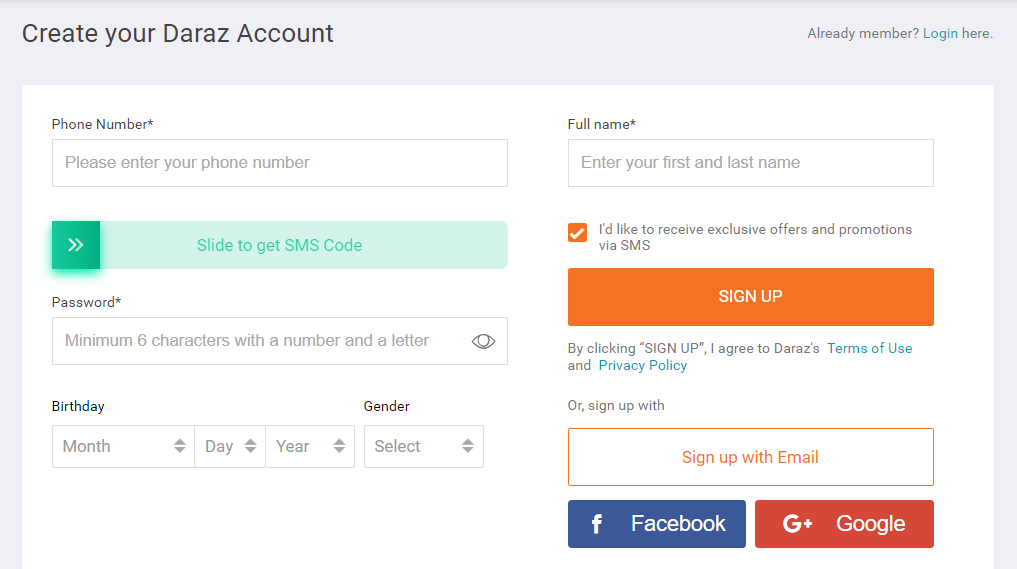This image is a screenshot of the "Create Your Duraz Account" registration form, set on a white background framed with a gray border. At the top of the form, the header reads, "Create Your Duraz Account." Below this, there's a prompt for existing members that says "Already a member?" followed by a blue hyperlink stating "Login here."

The form fields include:
- **Phone Number**: An input box required for entering your phone number, marked with an asterisk.
- **Full Name**: Another required field indicated by an asterisk, with an associated input box.
- **Get SMS Code**: A green rectangle with a smaller green square slot within it, presumably a button to receive a code via SMS.
- **Password**: Input box for setting a password.
- **Birthday**: Input fields to select the month, day, and year.
- **Gender**: A dropdown menu labeled "Select."

There is also a checkbox that is checked by default, next to the text "I'd like to receive exclusive offers and promotions via SMS."

At the bottom of the form is an orange rectangle with the text "Sign Up" in white lettering. Below this button, there is a disclaimer in quotation marks that reads, "By clicking 'Sign Up', I agree to Duraz's Terms of Use and Privacy Policy," with "Terms of Use" and "Privacy Policy" as blue clickable links.

The form also offers alternative signup options:
- A red rectangle labeled "Sign Up with Email."
- Two additional red and blue rectangles for signing up with Google and Facebook respectively.